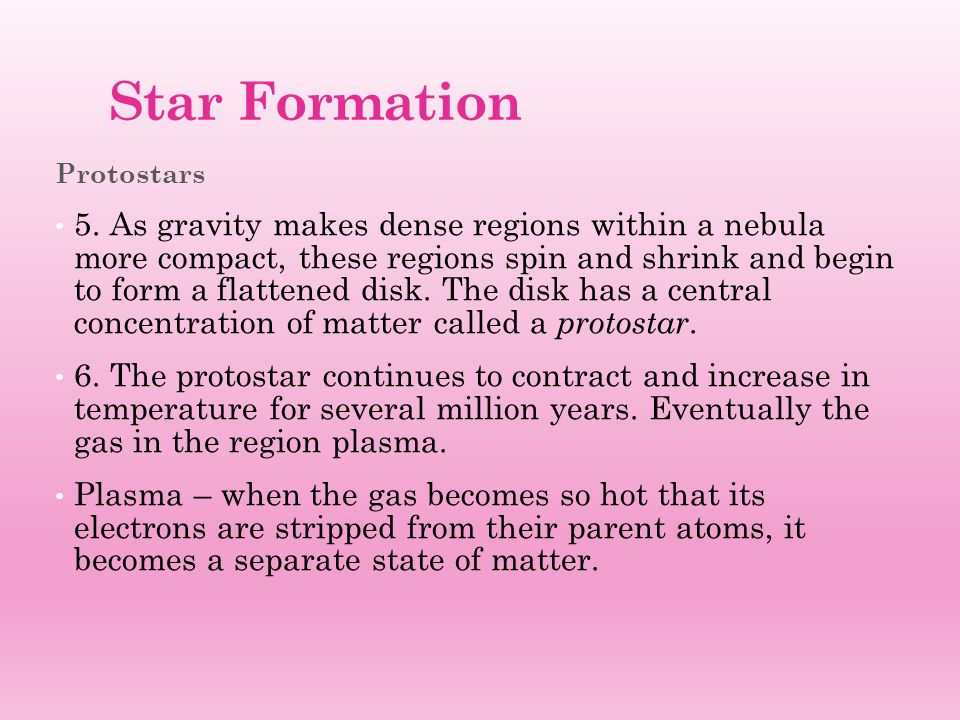The presentation slide features a gradient background transitioning from white to pink and back to white. At the top left, the heading "Star Formation" is displayed in pink text, followed by the subheading "Proto-stars" in grey text. Below, there are three bullet points numbered five and six, and an additional point on plasma, all in black text. Bullet point five explains that as gravity compacts dense regions within a nebula, these regions spin, shrink, and form a flattened disk with a central concentration of matter known as a proto-star. Bullet point six describes how the proto-star continues to contract and increase in temperature over several million years, leading to the formation of plasma. The third point elaborates that plasma occurs when gas becomes so hot that its electrons are stripped from their parent atoms, resulting in a separate state of matter. The slide is centrally positioned but slightly to the left on the page.